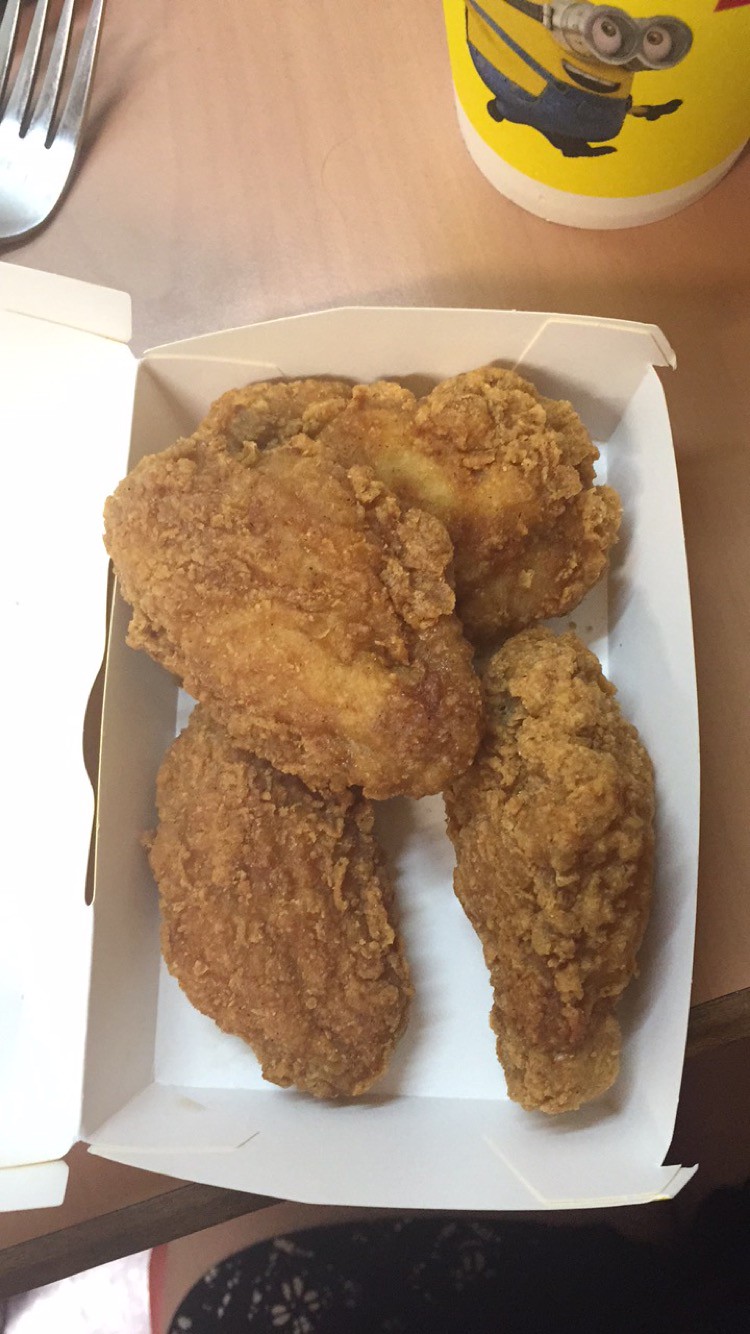This overhead, portrait-mode image captures a tantalizing meal of four golden brown pieces of fried chicken arranged in a white cardboard serving container atop a light faux wood table. The chicken includes two wings and two small breasts, all with crispy, fried batter detailing their delicious texture. In the top right corner, there is a partial view of a yellow cup featuring a Minion from the movie "Minions," identifiable by its blue overalls and signature metal glasses. The top left of the photo reveals just the tines of a silver fork. At the bottom of the image, part of a woman's lap is visible, displaying a blue dress adorned with a tan or white flower design and a glimpse of her knee. The overall scene sets a casual and appetizing dining atmosphere at a restaurant.